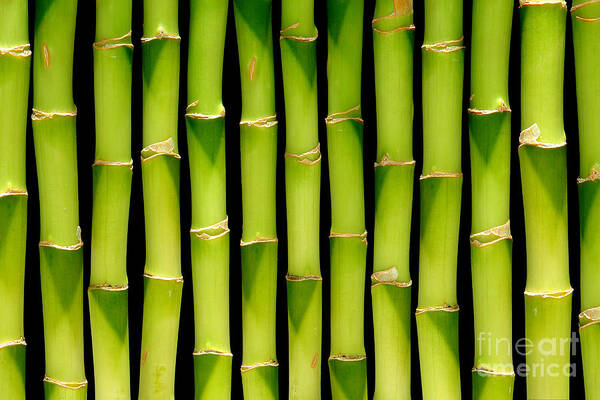In the image, we see a tightly zoomed-in shot of 13 vertical bamboo stalks arranged side by side, extending beyond the frame on both the left and right sides. Each bamboo stalk has multiple horizontal notches, with three or more on each piece, situated at varying heights. The stalks display a harmonious mixture of green, yellow, brown, and white hues, standing out against a solid black background. These color variations, along with the natural imperfections of the bamboo, add to the intricate texture and visual appeal of the composition. The bottom right corner of the image features faint white text that reads "Fine Art America." The overall setting gives a strong impression of nature, as the bamboo stalks dominate the image, leaving no other background elements visible.